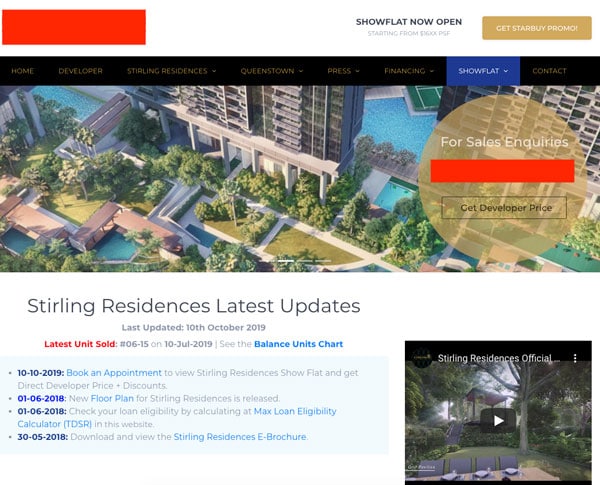Detailed Caption: 

The webpage presents a clean, modern aesthetic with a comprehensive navigation system. At the top left corner, a large, empty red rectangle provides a striking accent. Beneath this, a horizontal, black navigation bar spans the width of the page. The navigation menu items read: "Home," "Developer," "Residences," "Queenstown," "Press," "Financing," "Showflat," and "Contact," with most items featuring dropdown menus for detailed exploration. Notably, the "Showflat" tab is highlighted in blue.

Occupying the central portion of the page, a vibrant photograph displays a collection of high-rise condominium buildings surrounded by lush green spaces, creating a sense of contemporary urban living. On the right side of this image, a see-through brown circle invites users to make "Sales Inquiries."

Beneath the main image, another brown rectangle with a similar hue to the circular inquiry button beckons visitors to "Get Developer Prices." This button features a subtle brown outline and font, maintaining a consistent design theme. The semi-transparent nature of the brown circle allows the underlying photograph to remain visible, adding depth to the design.

Further down, the page provides critical information about the property, labeled as "Sterling Residences." The subheading "Latest Updates" indicates the most recent activity, noting the page was last updated on October 10, 2019, and also lists the latest units sold.